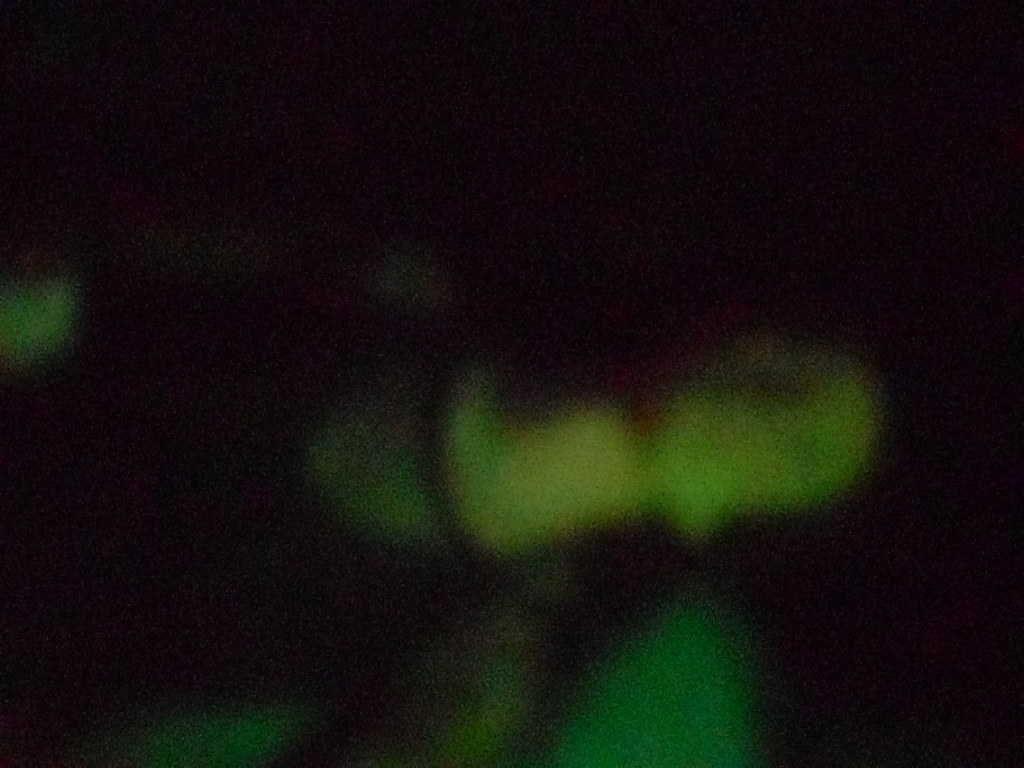In this abstract painting, the majority of the image is dominated by a pitch-black background, taking up approximately 70% of the space, reminiscent of the night sky during an Aurora Borealis. Amidst this darkness, faint but bright shapes in shades of green punctuate the scene, creating a striking contrast. Central to the image, slightly off to the right, is a thick, handlebar mustache-like form made of blurred, overlapping green hues, echoing the chaotic beauty of the Northern Lights with hints of yellow and green. Below this central shape, three pointed, fuzzy-edged green protuberances, resembling leaves, emerge. The two outer leaves are a bright grass green while the middle one is a darker lime green, connecting to a horizontally oriented cylinder that suggests a flower pod. The image is very blurry and pixelated, with indistinct shapes contributing to an overall mystical and dreamlike quality.